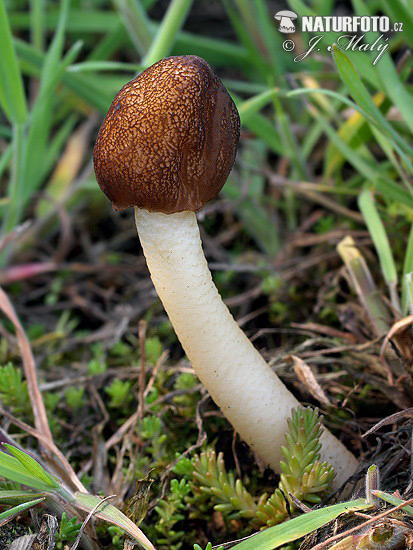This close-up photograph captures a young mushroom sprouting from the ground, positioned towards the bottom right and curving gently to the left as it ascends towards the middle of the image before the cap tilts slightly to the right. The mushroom features a pale white stem and a dark brown cap adorned with subtle white speckling. The setting is rich with detail; the mushroom emerges from a bed of leaf litter and twigs, surrounded by vibrant green grass and possibly some moss leaflets. The background includes more twigs and green leaves, slightly out of focus, while sunlight subtly filters through, suggesting a late-evening ambiance. In the upper right-hand corner of the image, the text "naturephoto.cz" appears alongside the photographer's signature, "J. Mally" (with an accent over the 'Y'), accompanied by a small mushroom logo, indicating that this image is part of a mushroom-themed collection.